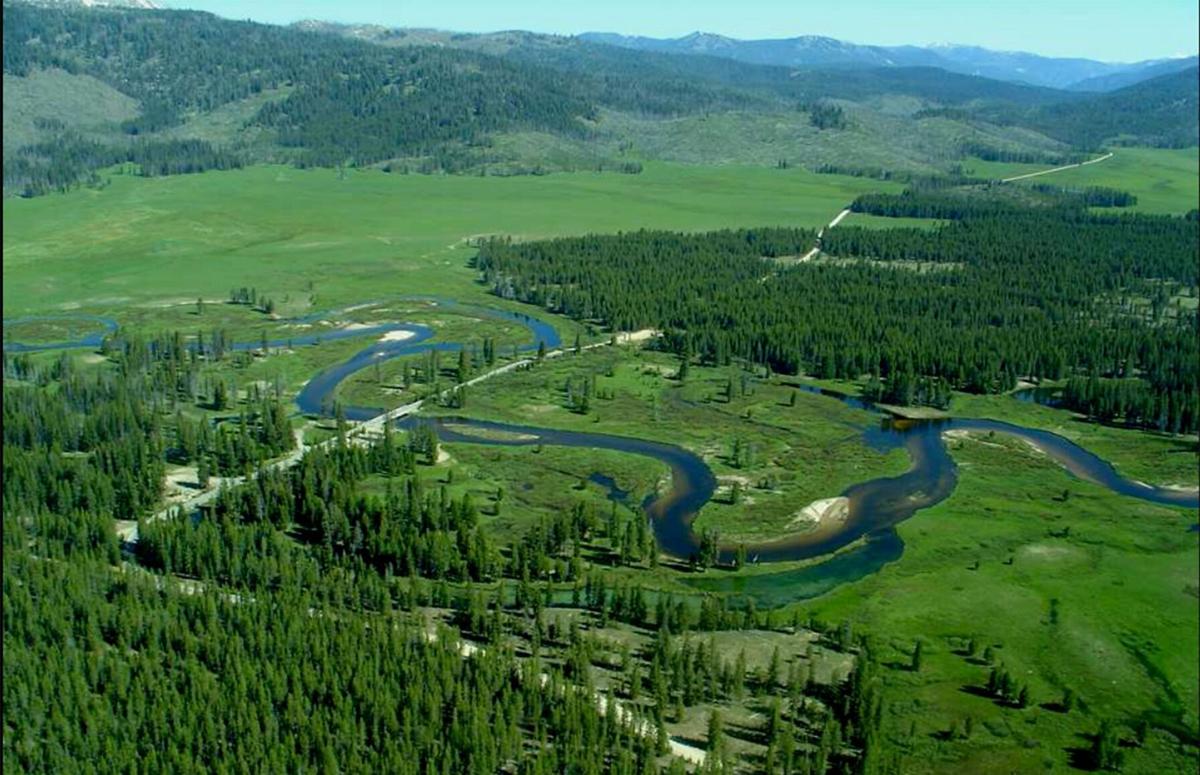The photograph is a wide, rectangular, aerial shot, likely taken from a helicopter or the top of a mountain, capturing a sprawling, scenic landscape. In the foreground, a lush expanse of flat land is dotted with tall, dark green pine trees and covered in lighter green grass. A winding river, dark bluish-black, snakes horizontally through the center of the image, evoking a sense of unyielded natural flow. To the right, a tan road runs slightly vertically, fading amidst the trees and extending into the distance. On the right side, a bridge crosses the river, connecting patches of forest on either side. The background reveals hills and mountains, painted in bluish-gray tones and capped with more pines, leading up to a very light blue sky that forms a serene backdrop to the vivid landscape below.